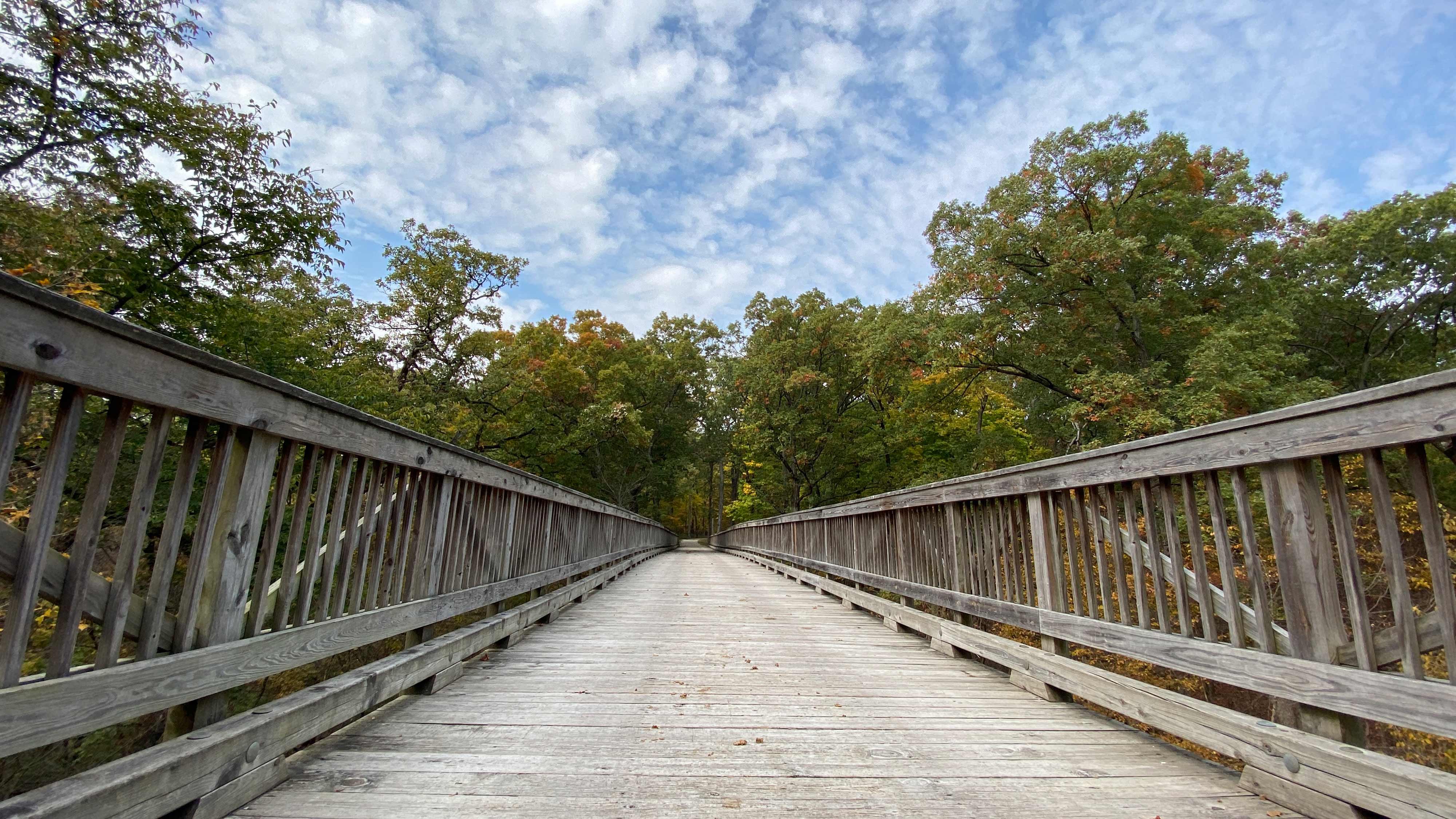The image features a weathered wooden bridge, displaying a mix of brown and gray hues. The bridge is relatively wide, with railings on both sides, leading deep into the picture and disappearing into what seems to be a gray trail. Flanked by tall and vibrant green trees, the scene suggests a transition from summer to early fall, evidenced by some leaves turning yellow, orange, and even a hint of reddish. The sky overhead is a bright blue adorned with broken, wispy white clouds, adding to the well-lit, sunny ambiance of the scene. Overall, the picture captures a natural, serene setting, emphasizing the bridge as a path cutting through the lush foliage.